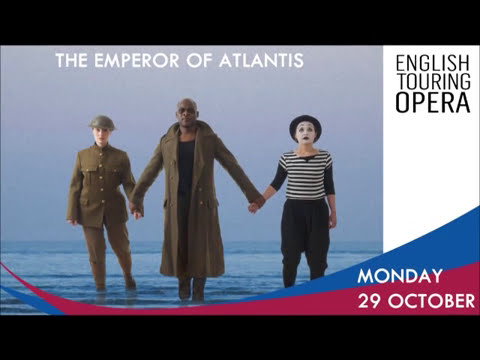The image is an advertisement for an opera entitled "The Emperor of Atlantis." At the top left, in bold white letters, it says "The Emperor of Atlantis." Below, three distinct characters emerge from an ocean. From left to right: a World War I soldier, wearing a metal helmet and gray army attire; a black man in the center, sporting dark sunglasses, a long brown trench coat, and black clothes, resembling a character from The Matrix; and a mime on the right, dressed in a black and white striped shirt with a painted white face, black hat, and black pants. These figures are walking on water, creating a surreal visuals. In the top right corner, it reads "English Touring Opera." The bottom right corner mentions the date, "Monday, 29 October." The overall composition and attire of the characters suggest a blend of historical and contemporary influences, promoting an intriguing and modern production of the opera.